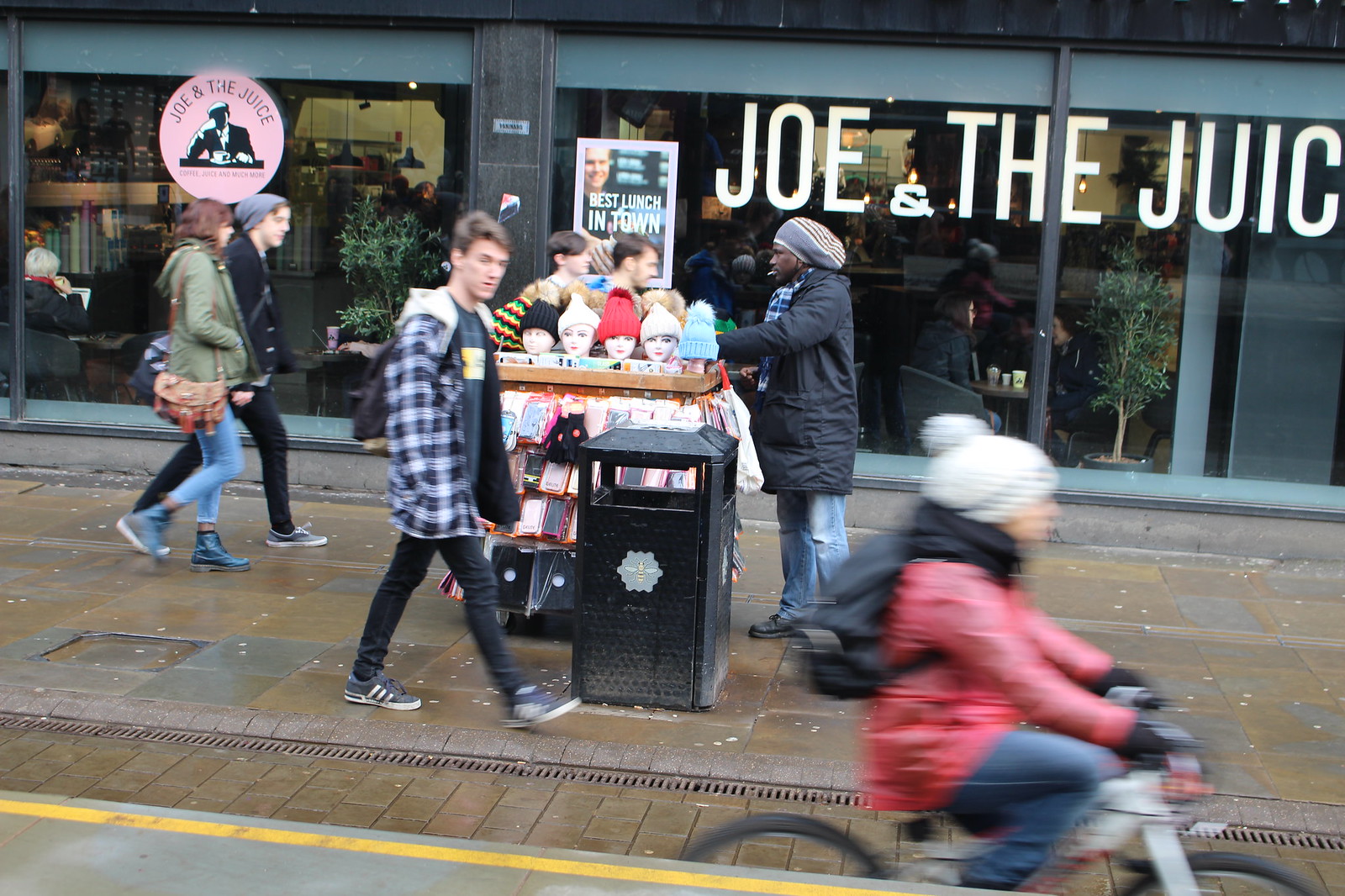The image captures a bustling outdoor street scene on a wet, brown stone sidewalk, likely due to recent rain. In the foreground, a person wearing a red raincoat and white hat rides a white bike swiftly through the scene, making them appear slightly blurry. To the left of the cyclist, a street vendor stands beside a trash can, overseeing a cart adorned with mannequin heads showcasing various hats, including black, white, red, and blue beanies. The vendor himself wears a hat and is looking to the left.

In the mid-ground, several young pedestrians are walking along the sidewalk, with most appearing to head in the same direction. In the background, a building with large windows reveals an establishment named "Joe and the Juice." The signage is clearly displayed both within a circular logo on the left and written across the windows on the right. Inside the shop, patrons can be seen sitting at tables, enjoying their drinks amidst visible greenery. The entire scene is a vivid portrayal of urban life, with a mix of commerce, movement, and a hint of community.